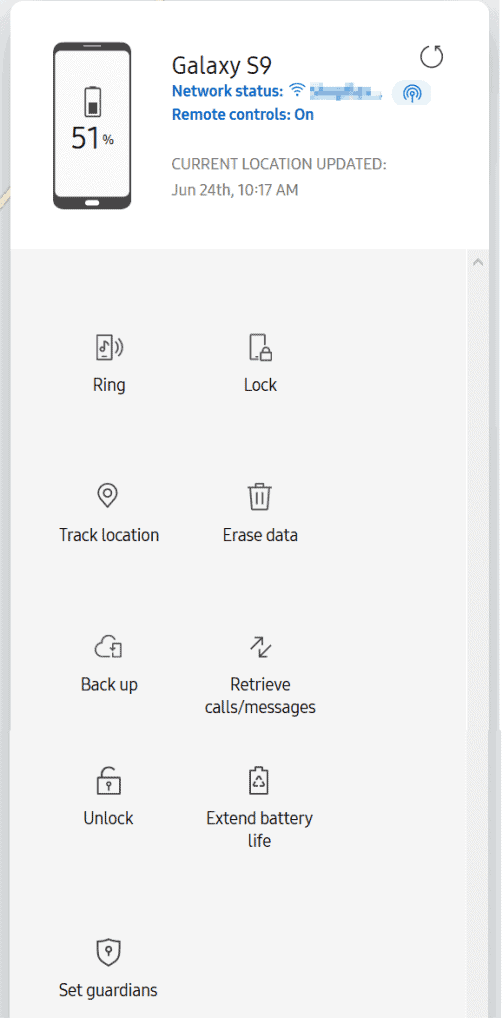The image features a smartphone interface with a light gray border on the left, top, and right sides. The borders on the left and right are significantly wider than the one on the top. At the top, there is a rectangular section with a white background displaying black text that reads "Galaxy S9." To the left of this text is an image of a smartphone showing a battery icon indicating 51% charge. Below "Galaxy S9," in blue text, it says "Network Status: Remote Controls On." Underneath that, in gray capital letters, it states "Current Location Updating." Further down, the date "June 24th, 10:17 AM" is displayed. The remainder of the background is light gray, featuring two rows of text on the left and right sides. On the left row, from top to bottom, the text reads: "Ring," "Track Location," "Backup," "Unlock," and "Set Guardians."